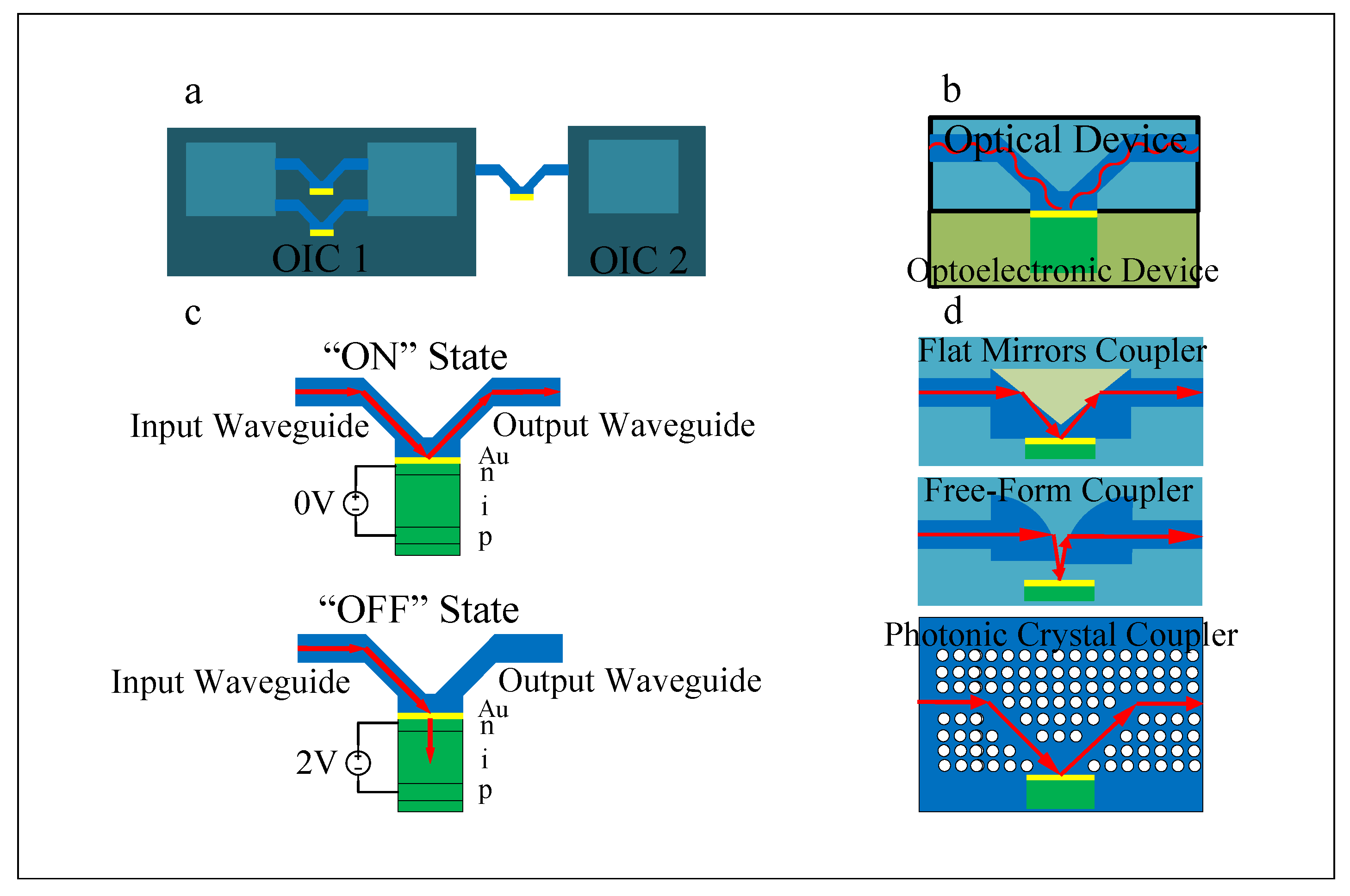The image is a detailed instructional diagram on an optical and optoelectronic device with sections labeled A, B, C, and D. 

**Section A** shows two blue rectangles labeled OIC-1 and OIC-2. OIC-1 has two lighter blue squares within it, connected by two bright blue lines with a yellow section at the bottom. Below these elements, it reads "OIC-1." A bright blue line with a yellow section at the bottom connects OIC-1 to OIC-2, which is represented as a dark blue square with a light blue square inside it, labeled "OIC-2."

**Section B**, positioned on the right side of the image, displays a blue square with blue and olive green sections, and green and blue components with red currents running through them. This section mentions "optical vice" and "optoelectronic device."

**Section C** illustrates diagrams of different states. The first diagram, labeled "on state," shows an input waveguide on the left and an output waveguide on the right, with blue sections and red currents running through them, along with a symbol for zero volts. Below that, the "off state" diagram shows the blue section splitting, with labeled input and output waveguides, and red currents again.

**Section D**, located in the lower right, consists of three diagrams of couplers. The top one, labeled "flat mirrors coupler," has a light blue background with a brighter blue section and red current arrows bouncing off a green and yellow rectangle at the bottom. Below it is the "freeform coupler" diagram, which also shows red current arrows bouncing off a structure at the bottom. The bottom-most diagram, labeled "photonic crystal coupler," shows red arrows and features white circles (polka dots) in the background, indicating complex interactions at the bottom.

The diagram is visually rich and detailed, ideal for someone with a background in electrical or optical engineering.